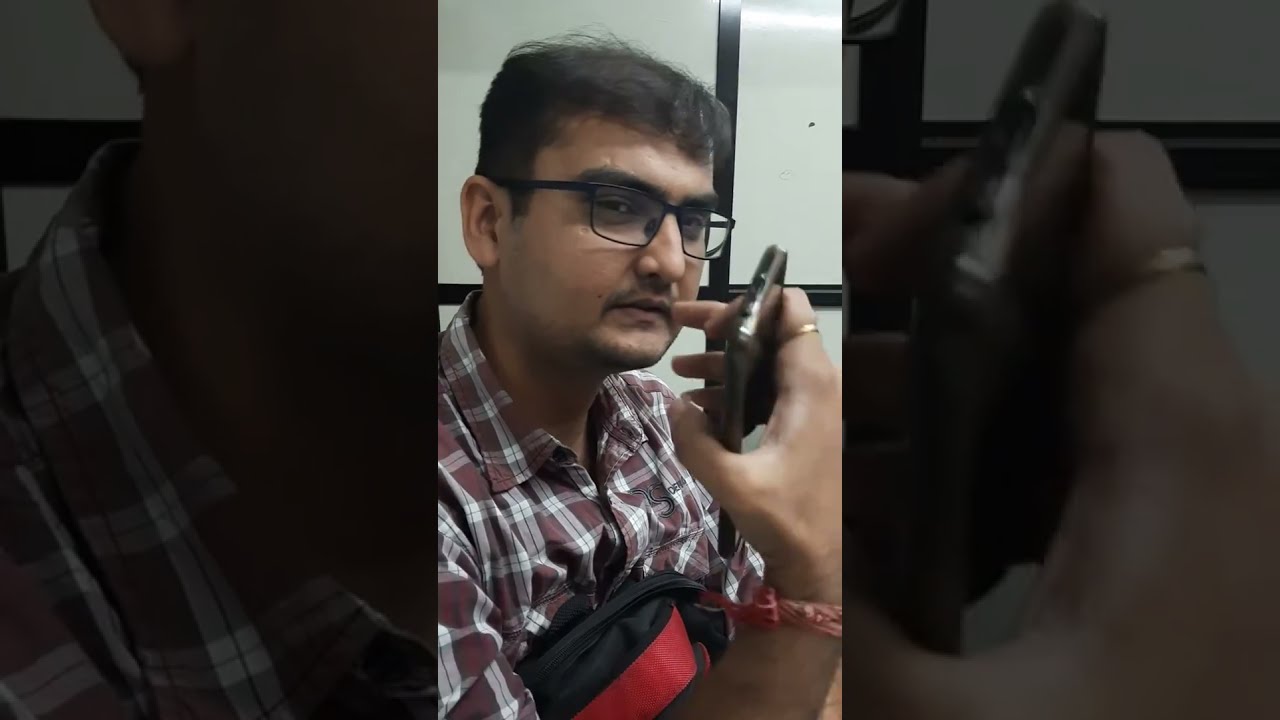This is a vertical, portrait-mode color photograph capturing a young man of Indian descent. He is seated at an angle, slouched slightly forward, with his head tilted to his right, smiling and looking directly at the camera, his teeth showing. He has short, somewhat thinning dark hair and wears black rectangular-framed glasses. His complexion is darker. He is dressed in a brown, maroon, and white plaid shirt. Clutched against his stomach between his arms is a black bag with a distinctive red stripe and thin red stitching. The background is a white wall with an overlaying black lattice framework. The image is framed by plain black bands on either side, emphasizing its tall and narrow orientation.